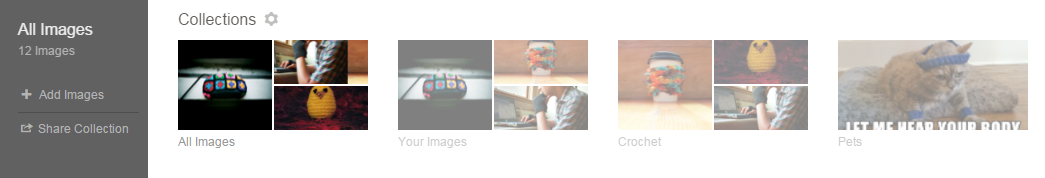The image showcases a detailed interface of a photo management system. Starting from the left side, there is a vertical gray rectangle with the heading "All Images" in bold white text at the top. Below that, non-bold white text reads "12 images," followed by a space, a plus sign, and the phrase "Add Images." A dark gray horizontal line spans the width of the interface, beneath which the text "Share Collection" appears.

Further down, the main background is white with a title "Collections" in gray. The interface displays three sections of images:

1. The first section titled "All Images," which is highlighted brightly, includes:
   - A picture of a yellow chicken.
   - An image featuring colorful balls.
   - A photograph of someone's arm.

2. The second section titled "Your Images," which is faded, includes:
   - The same image of colorful balls.
   - The same photograph of someone's arm.
   - A new image of a coffee cup.

3. The third section titled "Crochet," also faded, includes:
   - The coffee cup image.
   - The same photograph of someone's arm.
   - An image of a blue headband that resembles a hat.

On the far right, there is an image of a white meme text on a blue headband which humorously reads, "Let me hear your body," pretending that a cat is working out. Underneath the meme is the title "Pets" with a capital P.

This detailed description captures the layout and content of the image in the interface depicted.